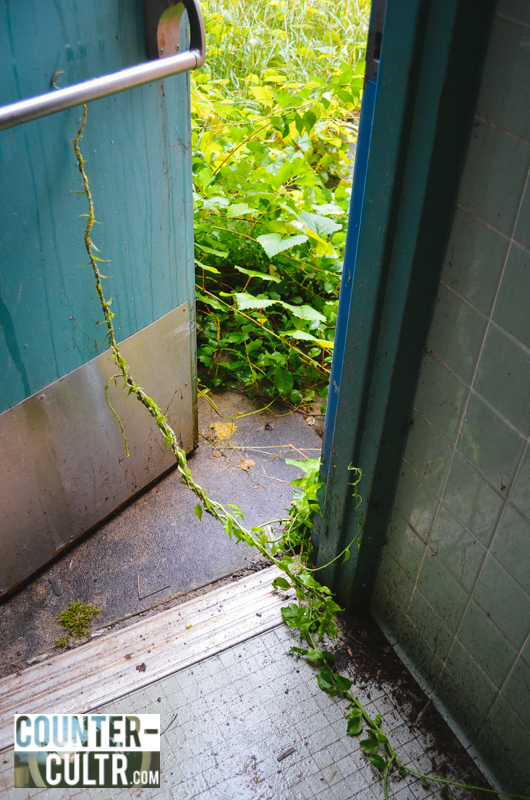The photograph captures an overgrown doorway, viewed from the inside of a building looking out. Dominating the scene is a partially open blue door, distinguished by a metal push bar and a silver kick plate at the bottom. The door appears old and weathered, with streaks of what looks like grease running down its surface. Through the open doorway, a vibrant vine winds around the push bar and extends into the building's interior, adding to the sense of nature reclaiming the space. The interior floors are made of very small square tiles, all heavily soiled and strewn with dirt and vegetation, suggesting long-term neglect. The wall to the right is lined with ceramic blue tiles, also smeared with mud, enhancing the overall feeling of decay. In the bottom left corner of the image, there is a logo that reads "counterculture.com".